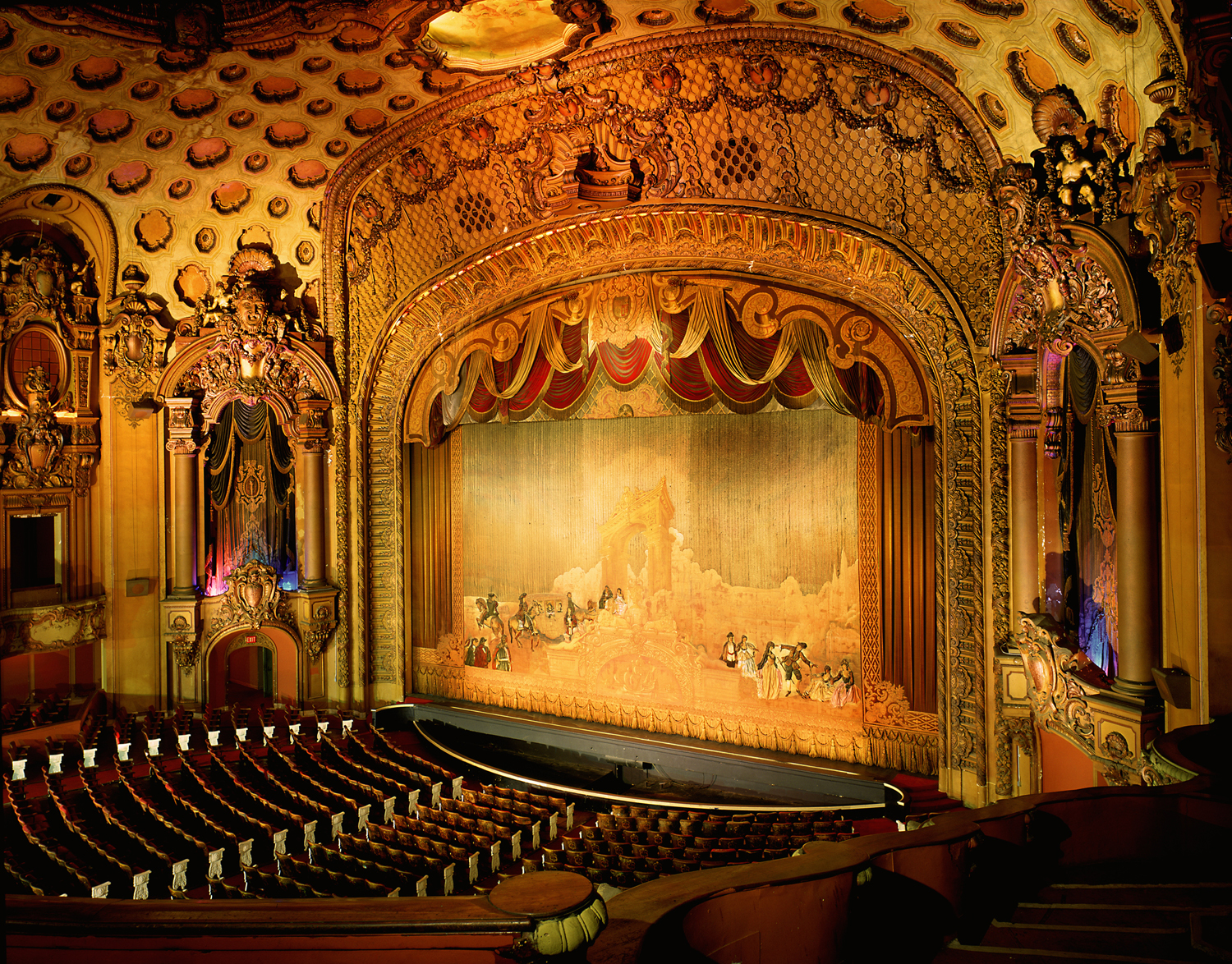This photograph captures the opulence of an old, grand theater, possibly an opera house, from an elevated balcony perspective, likely the second or first balcony. The rectangular image, approximately six inches wide and four inches high, showcases the intricate details of the venue. The foreground features a brown wooden banister, leading to a set of stairs on the right. The expansive, rounded stadium seating below appears to be in shades of brown and red, currently unoccupied. The stage area is concealed by a grand gold curtain adorned with an image of heavenly gates and groups of people, symbolizing a celestial scene. Above the stage, a striking red drape adds to the rich aesthetic. The theater's ceiling rises into a dome with circular recessed areas, painted in luxurious tones of gold, bronze, light brown, and red, underscoring the Baroque-style ornamentation that pervades this elegant space. The surrounding balconies and detailed decor emphasize the theater's historical and artistic significance.